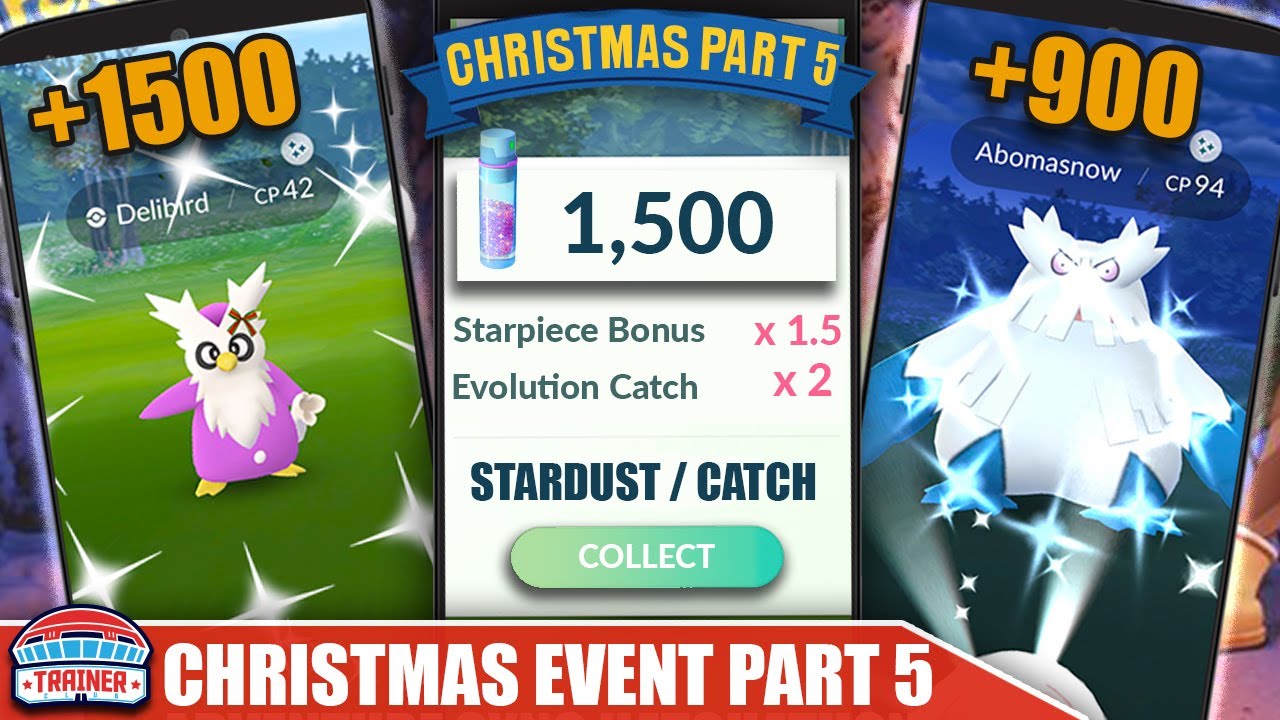The promotional image is divided into three distinct sections, each highlighting details of a special in-game Christmas event (Part 5) for a popular mobile game.

On the left side, there's an image of a smartphone displaying a bird-like creature labeled as Delibird with a Combat Power (CP) of 42. Above the creature's image, it indicates a bonus of +1500. Below the Delibird, some text reads "Christmas Part 5".

The middle portion of the image prominently features the text "Christmas Part 5" followed by details of event rewards. It states: “1500 Star Piece Bonus (x1.5), Evolution Catch (x2), and Stardust per Catch". There is also a large "Collect" button, inviting players to claim their rewards.

On the right side, there’s another section highlighting additional rewards. This part displays the text "+900" followed by a different creature labeled as Abomasnow with a CP of 94.

At the bottom left of the image, the text "Christmas Event Part 5" is reiterated, reinforcing the ongoing festive-themed event. 

The image overall is a vivid promotional snapshot aiming to entice players with special in-game bonuses during the Christmas event.